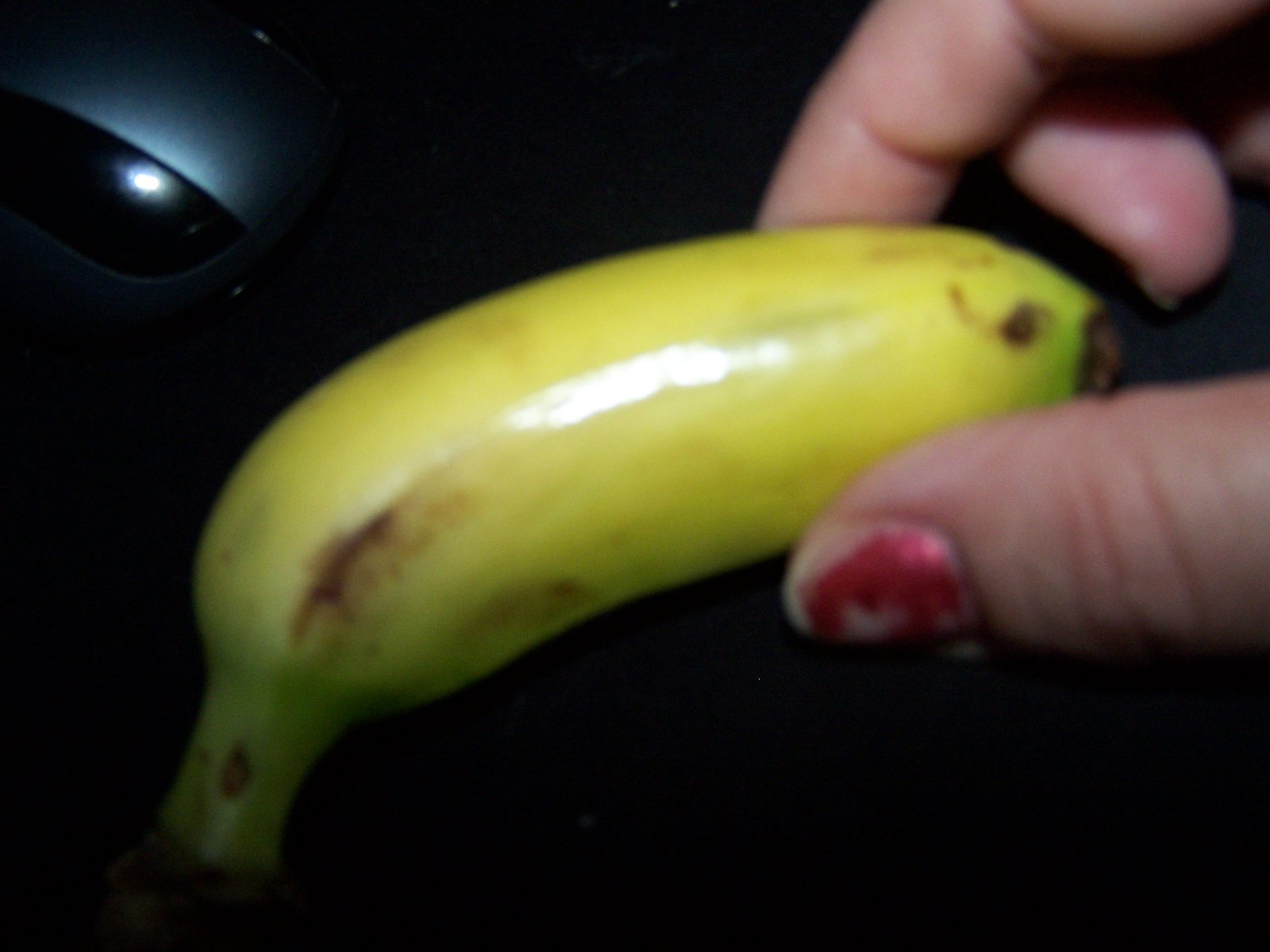In this image, we see a small banana held in a person's hand, set against an out-of-focus, blurry background. The photo appears to have been taken in a dimly lit room, and a bright flash was used, creating stark reflections on the objects. The person holding the banana has nails painted in metallic red, though the polish is chipped and peeling, showing signs of wear. The banana itself is not fully ripe, featuring green patches at the top and bottom, with the middle predominantly yellow and dotted with a few brown spots.

In the upper left-hand corner of the image, a computer mouse is faintly visible, somewhat resembling a car headlight due to the lighting and blur. The flash's impact is evident as it highlights parts of the banana and the mouse, adding a stark contrast to the darker surroundings. This grainy and poorly lit image captures the central focus of the hand-held banana with a computer mouse subtly blending into the background.